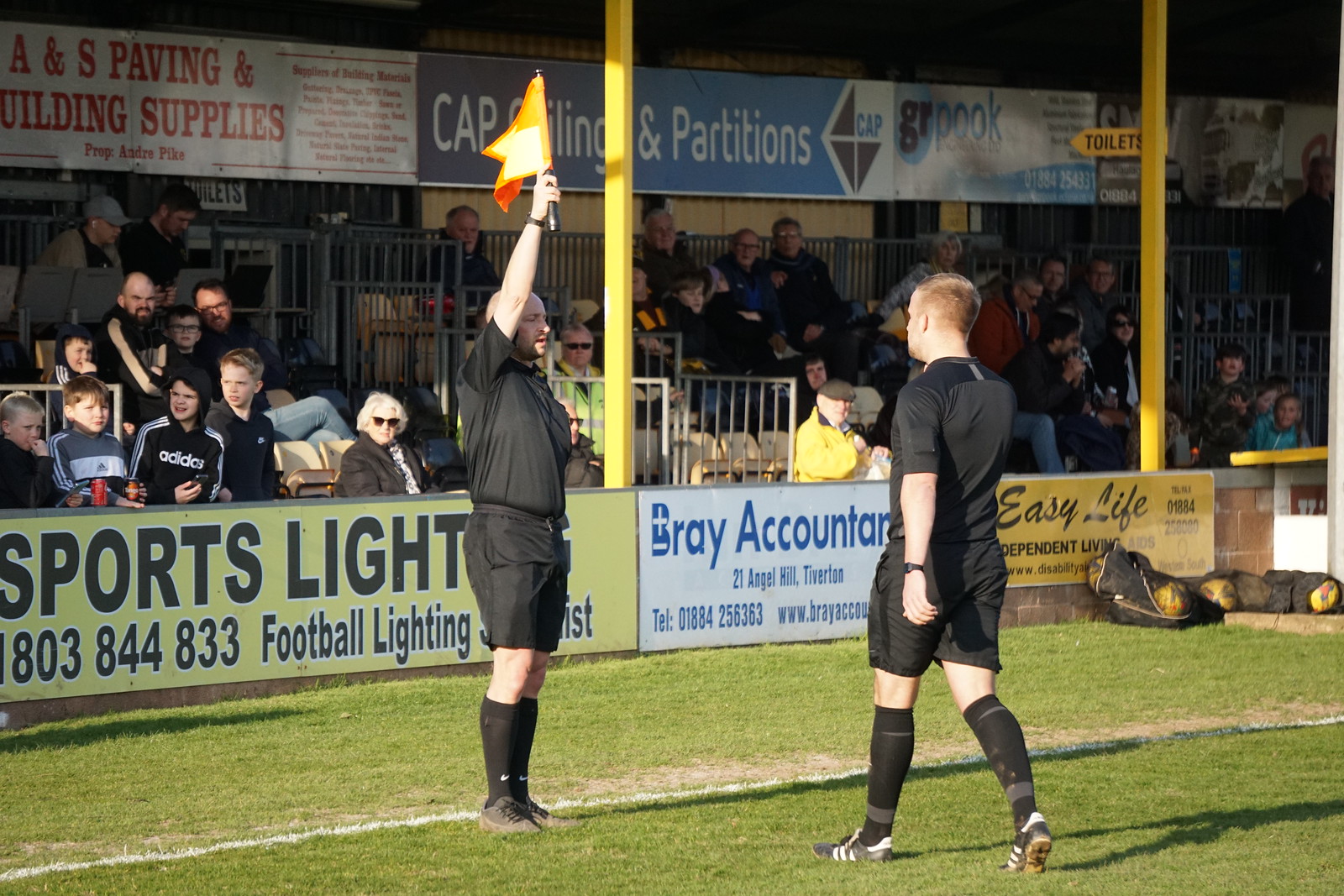This detailed photo captures a vibrant daytime scene on a lush green football field. In the foreground, at the edge of a white line, is a referee dressed in a black shirt, black shorts, and black socks, holding up an orange-yellow flag. Approaching him is a young man with light blonde hair, similarly clad in a black shirt, black shorts, and black socks, with cleats visible on his feet. Surrounding the field is a border lined with colorful advertising banners in yellow, white, blue, and red, featuring names such as "ANS Paving" and "CAP Filing Partitions." In the background, a crowd of spectators watches from the stands, draped in semi-darkness while the field remains brightly lit. The scene also includes several sports lights and poles visible above the stands, adding to the detailed ambiance of the football match in progress.